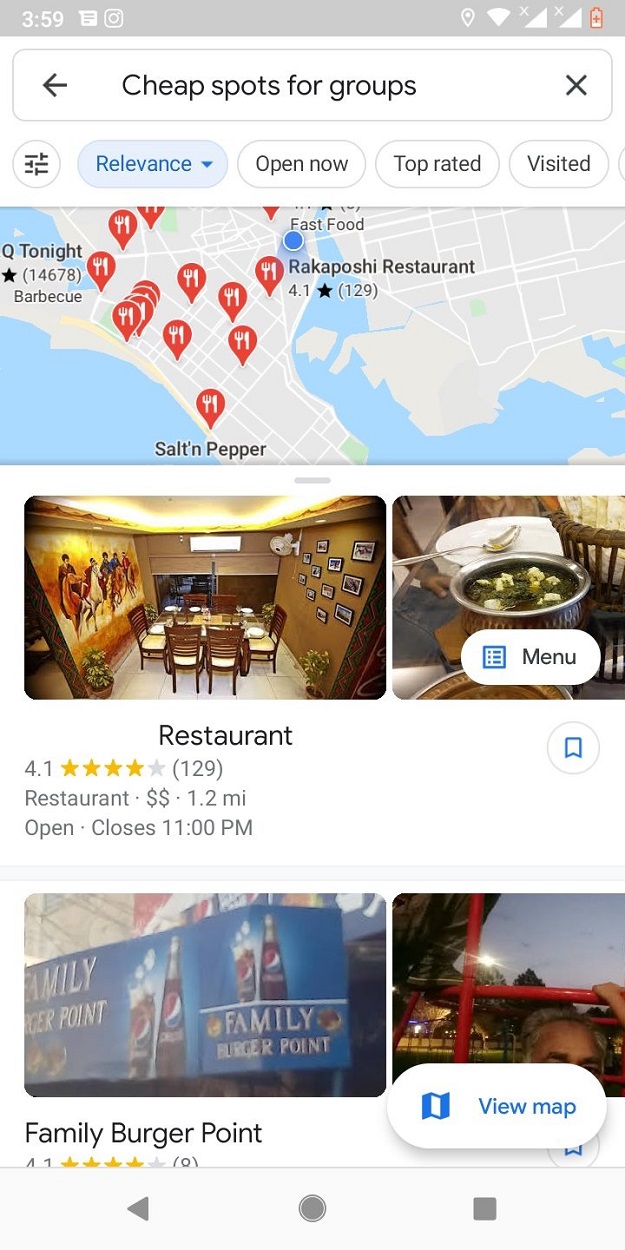This image appears to be a screenshot from a mobile device displaying a restaurant search result. The phone is resting on a gray surface, and the time shown on the screen is 3:59. There is a notification indicating low battery, highlighted in red, with a Wi-Fi connection but no cellular signal bars. 

At the top of the screen, there is a search bar labeled "cheap spot for groups," accompanied by a left arrow and an 'X' for clearing the search. Below this search bar, several filter buttons are visible: "Relevance" (highlighted in blue), "Open Now," "Top Rated," and "Visited" (all in white with black text, except "Relevance," which has blue text).

The screen further displays a map dotted with numerous red pins marked with fork and knife icons, signifying various restaurant locations. Below the map, the first search result features an image of a restaurant, indicating its rating as 4.1 stars based on 129 reviews, categorized as moderately priced with two dollar signs, located 1.2 miles away, and currently open until 11 p.m. Adjacent to this are more photos, where one displays "Menu" and another partially shows "Family Burger Point."

At the bottom of the screen, there is a button labeled "View on map," followed by the phone's navigation icons: back, home, and recent apps, colored in blue, gray, green, brown, and red respectively.